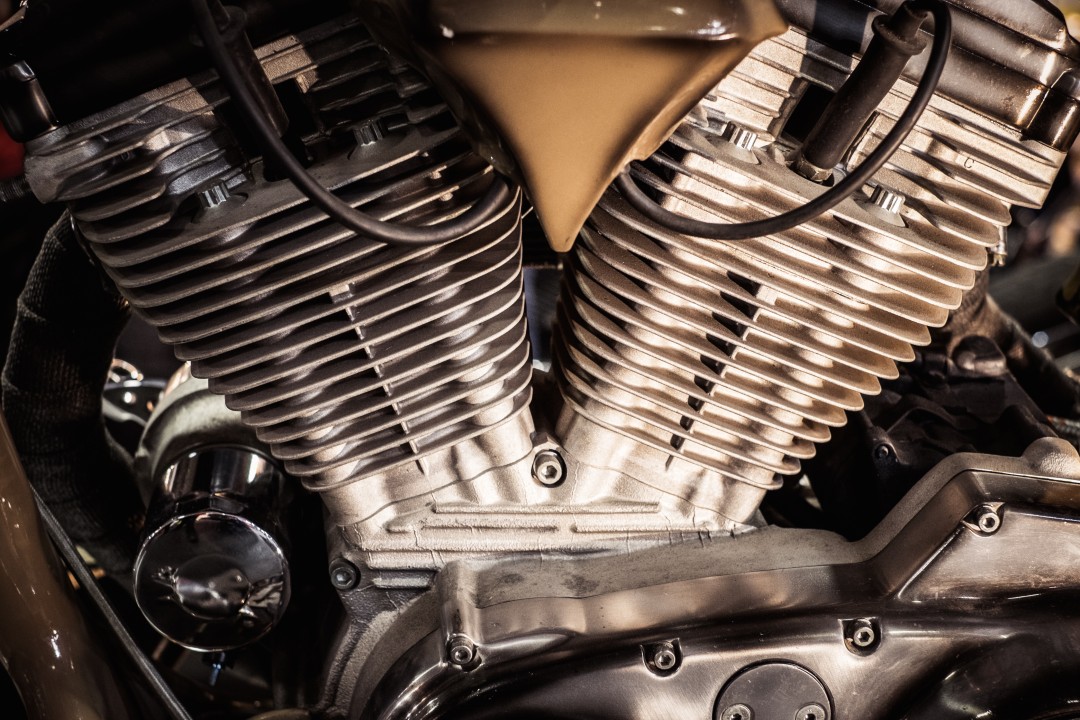This is a detailed close-up image of a mechanical gear or engine component, showcasing its intricate internal structure. The central focus is on two arm-like extensions made of shiny, silver metallic material, extending diagonally, one from the center to the upper left and the other from the center to the upper right. Both arms have black, rubber-coated wires plugged into them. The mechanism is surrounded by bolts and screws, and there is a polished, gold-painted metal section visible, adding a contrasting hue to the predominantly silver-colored parts. The overall appearance of the machinery is clean and well-maintained, with detailed, layered metal components resembling parts of a motorcycle engine or a similar machine. The lack of surrounding context emphasizes the inner workings of this complex mechanical assembly.